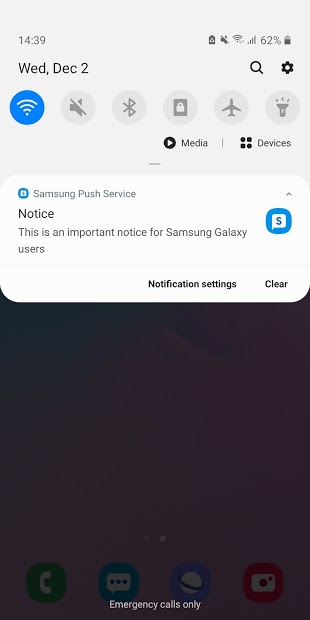Screenshot of a smartphone screen in portrait mode, displaying various elements with detailed descriptions:

At the very top of the screen, backed by a gray background, are the notification indicators. On the right-hand side, there are icons for the Wi-Fi signal, service signal, and battery level, while on the left-hand side, the time is displayed.

Below this gray bar, a black strip shows the date, "Wednesday, December 2nd." Adjacent to this on the right-hand side are a search bar and an options cogwheel.

Next, a blue Wi-Fi symbol is displayed, leading into more gray-backed status icons, including a volume indicator, a Bluetooth symbol, a lock within a square, an airplane (indicating airplane mode), and a flashlight icon.

Underneath the lock icon, the word "Media" appears in black text with a play button next to it. Below the flashlight and airplane icons, the word "Devices" is displayed alongside four black circles and squares.

Farther down, transitioning to a white background, a notification reads, "Samsung Push Service." This is followed by a bold text emphasizing the importance: "Notice: This is an important notice for Samsung Galaxy users." Accompanying this text is a blue 'S' within a word bubble, resting on a larger blue circle.

Below this notification, still on a white background, the options "Notification settings" and "Clear" are available in gray text.

Further down, the screen shows a heavily grayed-out view of the phone's interface, making details difficult to discern. At the bottom of the screen, phone icons are barely visible with the text, "Emergency calls only," highlighted in white.